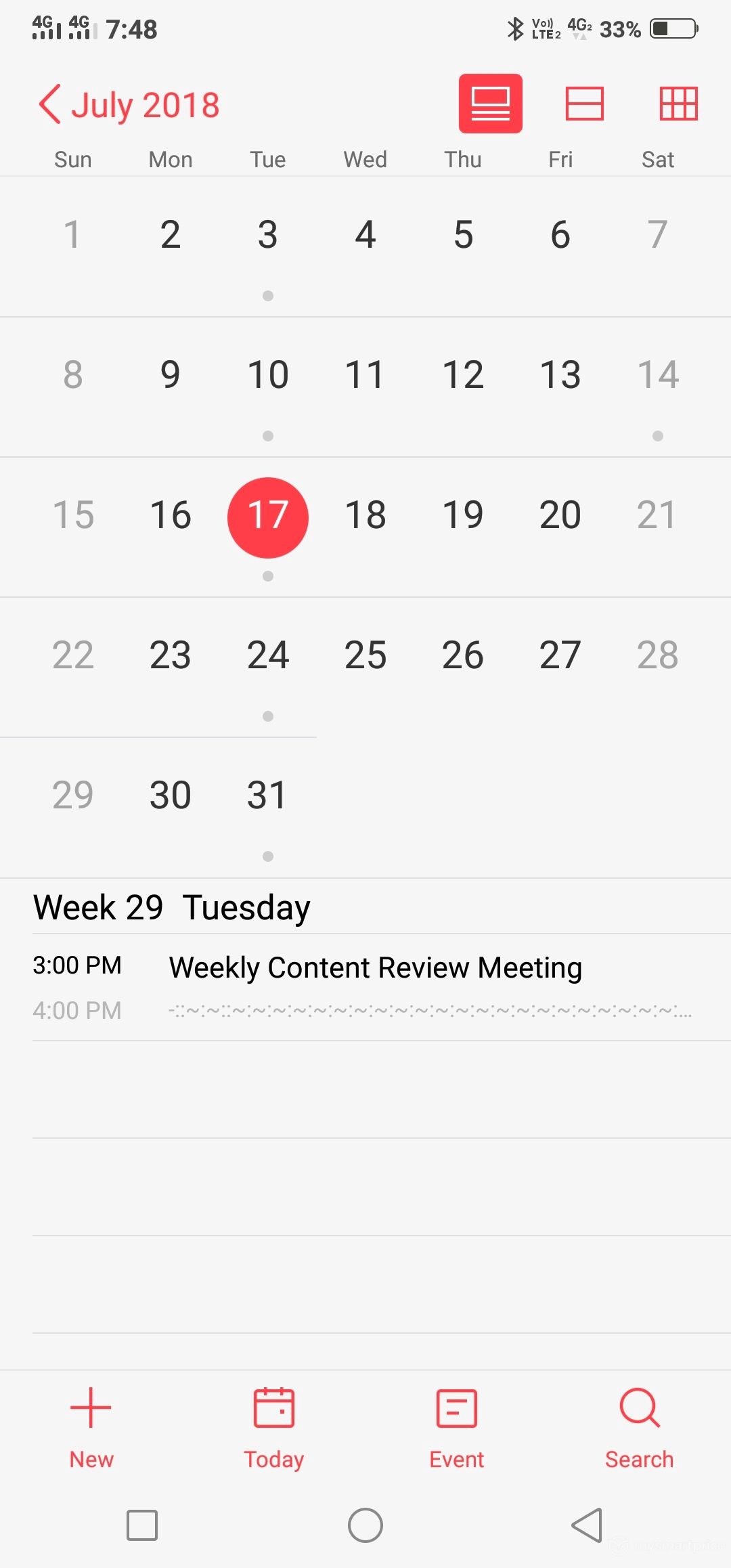The image appears to be a screenshot from a smartphone displaying a calendar app. In the top left corner, the screen indicates a 4G connection, with four signal bars next to the first 4G icon and three bars next to the second 4G icon. The time shown is 7:48, and the battery level in the upper right corner is at 33%.

The calendar is set against a gray background, and in the upper left, it is labeled "July 2018" in red text. The layout starts with Sunday the 1st in the upper left corner and goes through to Tuesday the 31st in the bottom right corner. Certain dates are marked with dots indicating saved items or events: the 3rd, 10th, 14th, 17th, 24th, and 31st of July. The date 17th of July is highlighted with a red circle, suggesting an important event.

At the bottom of the screen, it indicates "Week 29," with a specific event listed for Tuesday at 3 p.m.—a weekly content review meeting. There is an indication of another event at 4 p.m., though the text is cut off and not fully visible. 

The bottom of the screen includes several navigation options: a red plus sign labeled "New," a calendar icon labeled "Today," a square icon labeled "Event," and a magnifying glass icon labeled "Search."